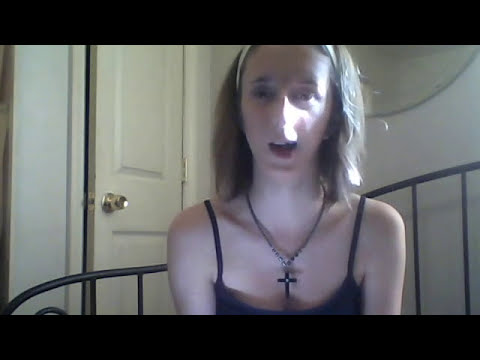This image is a still taken from a webcam, capturing a woman seated on her bed. The bed features a wrought iron frame with a distinctive design—a curved arch running upward to the right, accompanied by vertical bars. Behind her, there is a door slightly ajar with a gold handle, painted in off-white. The woman, positioned at the center of the image, appears to be mid-conversation, her mouth slightly open. She is wearing a black tank top, a necklace with a cross pendant, and a white headband that holds back her shoulder-length, dirty blonde hair. Light is streaming through a window, illuminating her nose and the right side of her face. The image has black bars at the top and bottom, emphasizing the central focus on her. The walls of the room are white, and some additional objects and details, including something hanging on the wall, are partially visible but cut off from view.